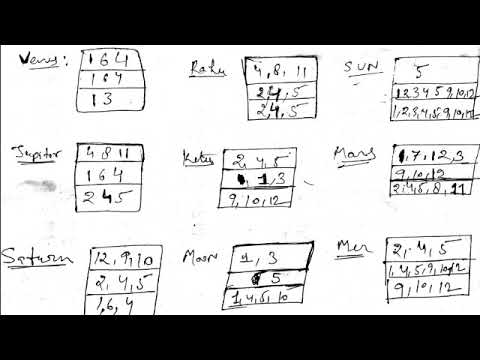The image is a black-and-white photograph depicting a handwritten grid of planetary data on a white background. The text is written in what appears to be black marker or pen. There are several rows, each labeled with the names of celestial bodies, including Venus, Jupiter, Saturn, Mars, Sun, Moon, and Mercury. Each row consists of a word underlined and accompanied by a box divided into three columns and three rows, containing multiple numbers.

For instance, the box labeled "Venus" contains the numbers 164 at the top, 164 in the middle, and 13 at the bottom. Other boxes feature numbers like 4811, 245, and 12, although some labels are difficult to decipher due to the handwriting. The box for the Sun contains a notable density of numbers, including 1, 2, 3, 4, 5, 9, 10, and 12. Each grid appears to represent some form of data classification related to the respective celestial body.

Overall, the image resembles a scientific or educational note where numerical data about planets and other astronomical objects are organized in a structured, albeit somewhat unpolished, format.